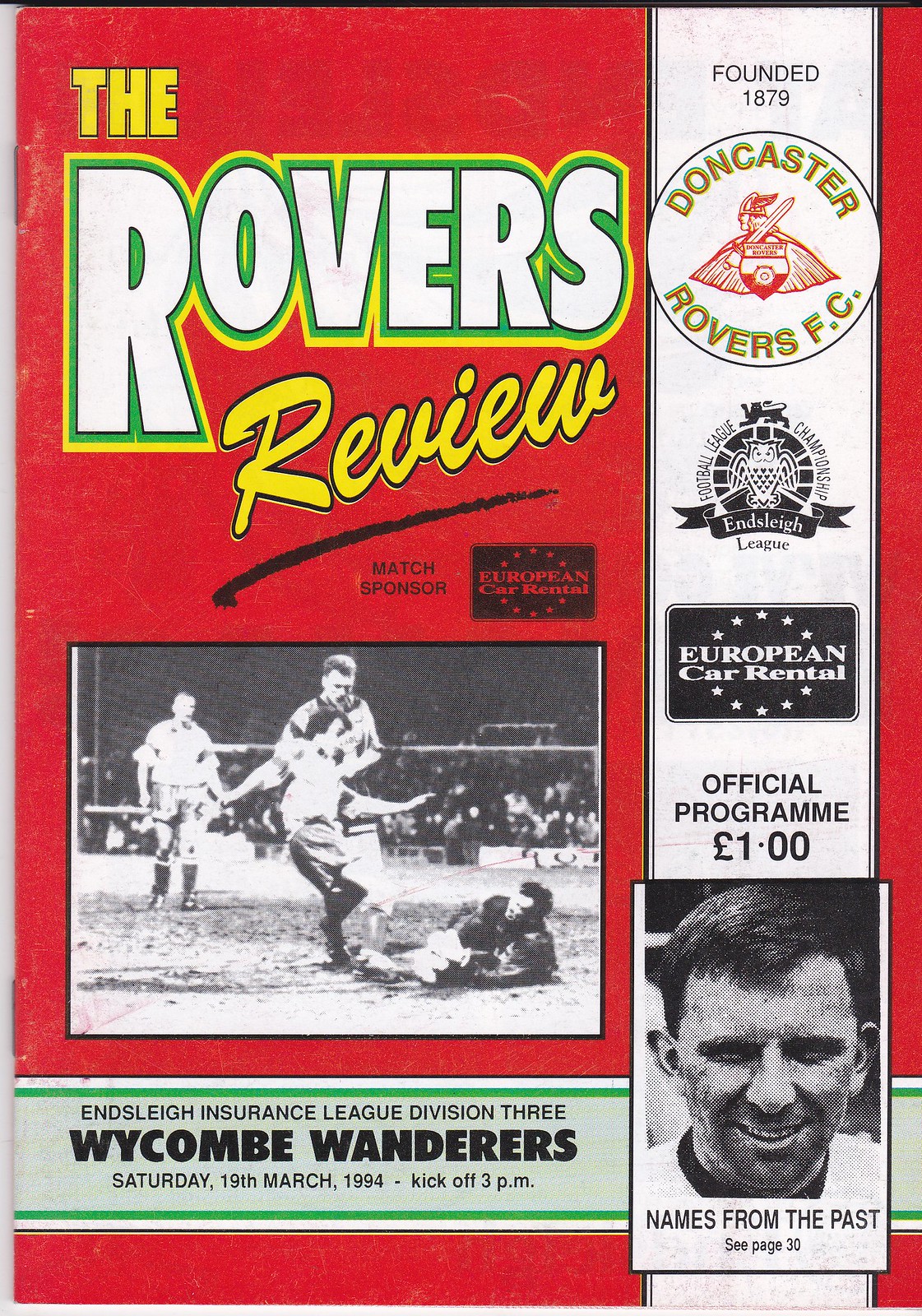The image shows a predominantly red magazine cover titled "The Rovers Review." The title is prominently displayed across the red background, with "The" and "Review" in yellow and "ROVERS" in white with a green outline. The word "ROVERS" is in all capital letters, while "Review" has only the "R" capitalized. There's a black, upside-down check mark beneath the title, followed by the text "Match Sponsor: European Car Rental."

Below this, the cover features a black-and-white photograph of a soccer game: one player is running with his right leg raised near a soccer ball, another player on the ground appears to be reaching for the ball, a third player watches the action, and a fourth player stands by with his arms at his sides. 

A vertical white banner runs down the right side of the cover, containing several pieces of information: "Founded 1879," "Doncaster Rovers FC," and "European Car Rental Official Program, One Pound or One Euro." At the bottom right corner, there's a photo of a smiling man with his hair swept from right to left and prominent ears. Next to this image, it reads "Names from the Past, see page 30."

At the bottom of the image, a green strip indicates additional details: "Inslee Insurance League Division 3 Wycombe Wanderers, Saturday 19th of March 1994, Kickoff 3 PM."